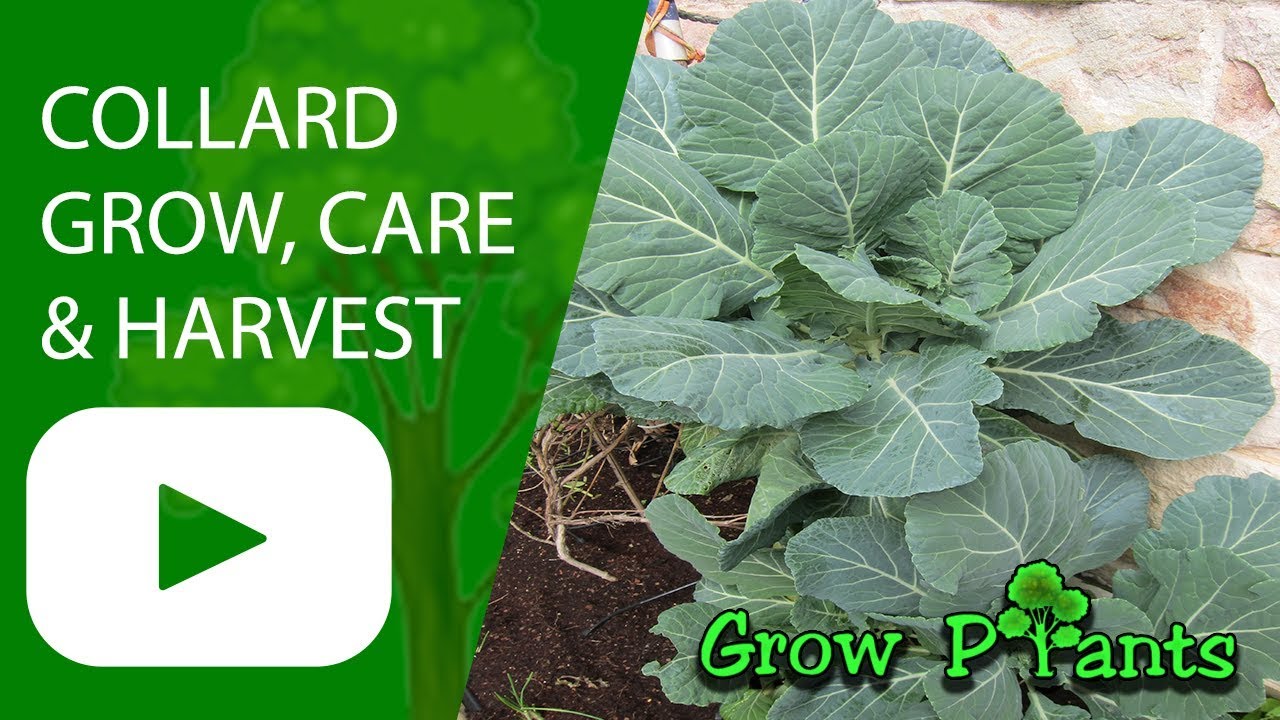The image displays a thumbnail for a YouTube video about gardening. On the left side, there's a stylized green background with a silhouette of a tree, overlaid with large white text that reads "Collect, Grow, Care, and Harvest." Below this text is a white YouTube logo. On the right side, there is a vibrant image of a green cabbage growing in brown soil, placed in front of a stone wall that has a light pinkish tint. At the bottom right corner of the image, the words "Grow Plants" are written in a stylized green font with a black drop shadow, and the letter "L" in "Plant" is creatively shaped like a plant. The entire thumbnail is designed to visually promote a gardening-themed video, emphasizing the steps in cultivating cabbage.